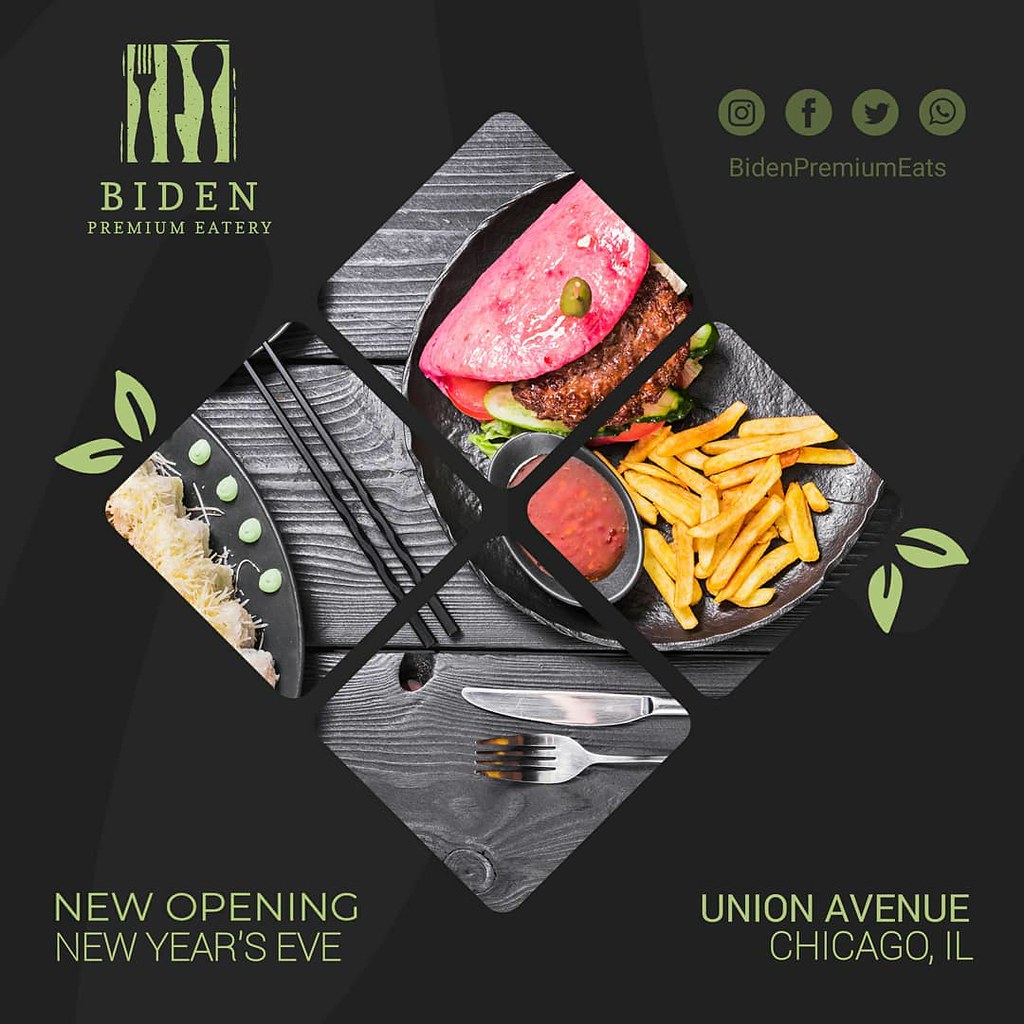This detailed image appears to be an advertisement for a new dining establishment. In the top left corner, it reads "Biden Premium Eatery," accompanied by a logo featuring a fork, knife, and spoon silhouette on a green cutting board. In the center of the image, a visually striking diamond shape is formed by dividing a square photo diagonally with black lines into four smaller diamond sections. Depicted in these sections is a top-down view of a wooden table laden with an assortment of food: a pan with grilled ham, a hamburger, French fries, dipping sauce, and a bowl seemingly filled with cheeses; the table is also set with forks, knives, and chopsticks.

The photo's background includes illustrations of small leaves adorning its borders, contributing a fresh and organic feel. In the top right corner, the text "Biden Premium Eats" appears along with social media icons for Instagram, Facebook, Twitter, and WhatsApp. Significant event details are provided in green writing: the bottom left corner announces "New Opening, New Year's Eve," while the bottom right specifies the location as "Union Avenue, Chicago, Illinois." The thoughtful layout and detailed design indicate this image is purposefully crafted for social media platforms, aimed at generating excitement and anticipation for the restaurant's grand opening.